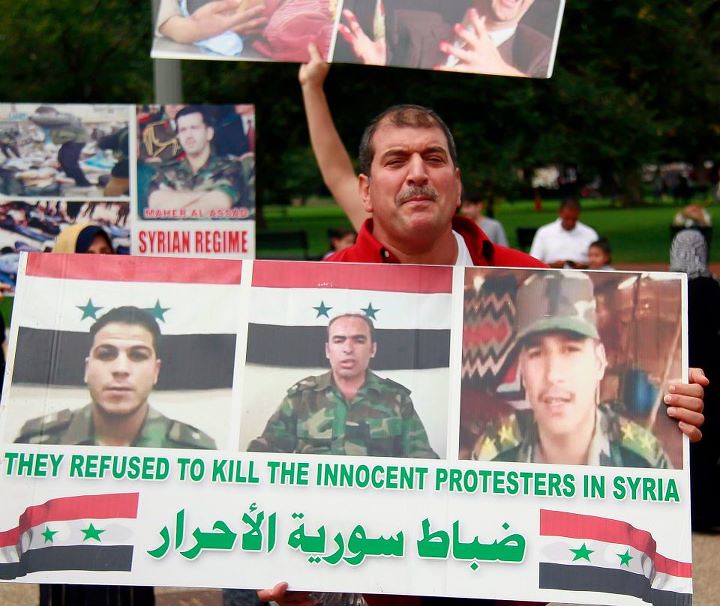In the image, we see a middle-aged man standing in a large grassy field, which appears to be a park, under the midday sun. The man, who has a mustache, dark brown hair with a receding hairline, and a tan complexion, is the central focus of the photograph. He is wearing a red collared shirt over a white undershirt and holds a large sign. The sign features three images of military personnel in camouflage uniforms, and prominently displays green text on a white background that reads, "THEY REFUSED TO KILL THE INNOCENT PROTESTERS IN SYRIA." Below the text are two flags, each split into horizontal thirds of red, white, and black stripes with two green stars on the white stripe. There is also text in a foreign language, likely Arabic, written in green. 

The background reveals several other protesters, some holding signs related to the Syrian regime, and milling about the park area. The surrounding scene is lush with green grass and trees, emphasizing the outdoor setting. The scene captures a moment of protest against the Syrian regime, with the man's emotional expression adding to the atmosphere of urgency and advocacy.